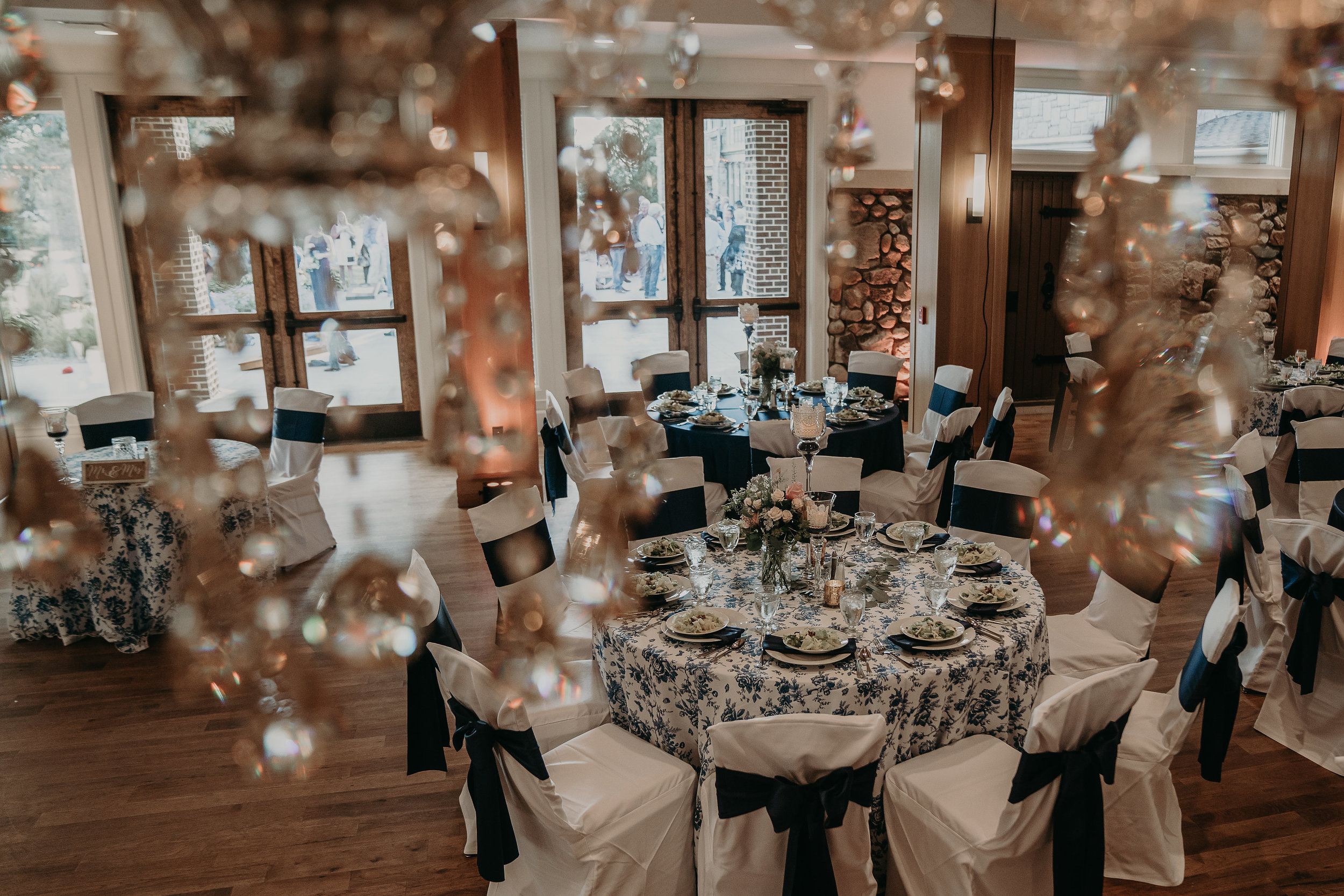This image captures an elaborate dining space, likely within a room in a house, restaurant, or furniture store. The horizontal rectangular frame showcases a central round table adorned with a blue and white floral-patterned tablecloth. The table is meticulously set, surrounded by ten chairs draped in white covers with black ribbons tied around them. Each place at the table includes a plate, a bowl with a napkin inside, totaling ten complete settings.

The polished wooden floor reflects the room's extensive decorations. Hanging ornaments from the ceiling and abundant wall decorations contribute to the room's ornate aesthetic. There are five tables in total within the image, all uniformly set. The photo appears to be taken from an elevated perspective, adding an interesting angle that highlights the room's decor and arrangement. In the background, two doors are visible, with possible silhouettes of people behind them, adding a subtle depth to the scene. This well-lit and detailed image presents a visually rich and inviting dining area.